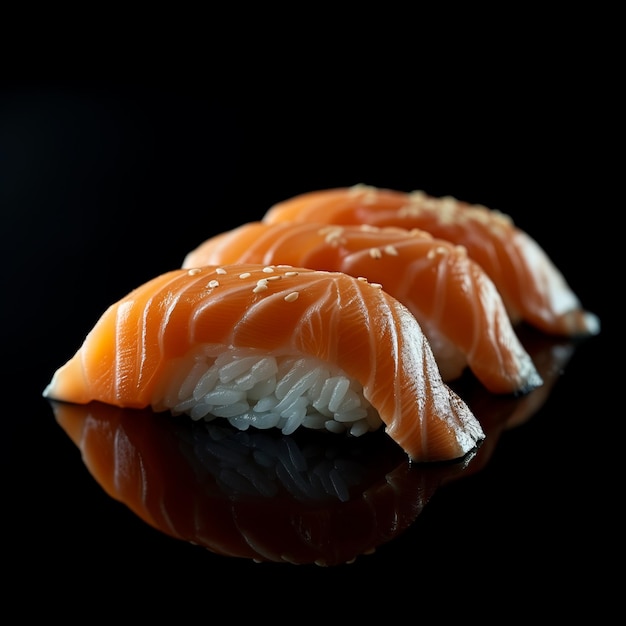In a close-up, square macro image, three pieces of salmon sashimi rest elegantly atop beds of white, sticky rice on a sleek, black surface. The salmon, a deep orange-pink hue, is generously sprinkled with sesame seeds. Approximately 30 grains of rice are visible beneath each piece of fish, which completely covers the rice from above. The glossy tabletop beneath reveals a subtle reflection of the sashimi, adding depth to the composition. All four corners of the image are solid black, drawing the viewer’s eye to the vivid, almost mirror-like reflections of the sushi in the center. Additionally, there's a noticeable glare on the right side of each piece of salmon, enhancing their glistening appearance.